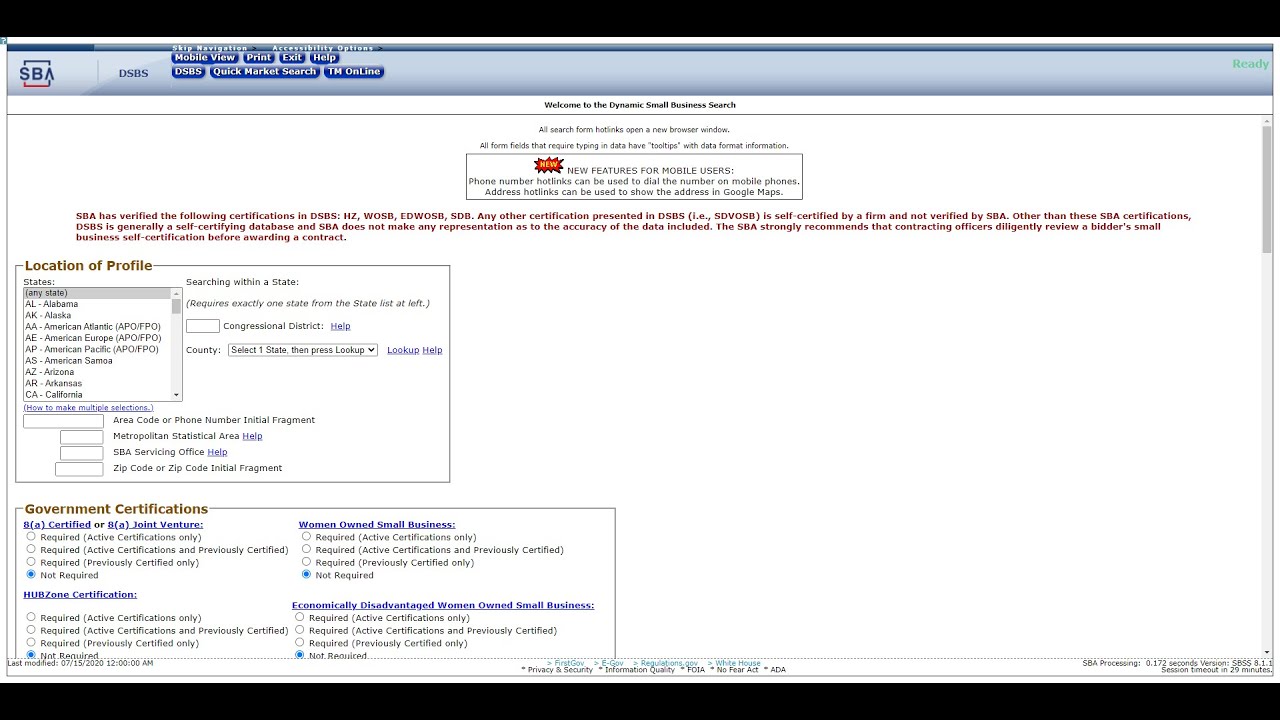In this image, we see a screenshot of a website primarily dedicated to assisting small businesses. The website features a logo in the top-left corner consisting of the letters "SB" followed by an upward-pointing arrow, which appears to symbolize growth or progress. To the right of the logo, the acronym "DSPS" is prominently displayed. Below this, a welcoming header reads, "Welcome to Dynamic Small Business Search."

The website contains multiple interactive elements, starting with a section labeled "All Search." This section lists various functionalities, including "Hot Links," and an option to "Open a New Browser Window." Additionally, it informs users that all form fields requiring data entry are equipped with tooltips providing data format information.

Further down, there is a box titled "Location and Profile," which includes options for selecting "States." Adjacent to this, another section named "Government Certifications" offers various certification options such as "8(a) Certified" or "8(a) Joint Venture," and "HUBZone Certification," among others. The comprehensive layout and finely detailed options suggest the website is a robust tool designed to support the needs and certification processes of small businesses.